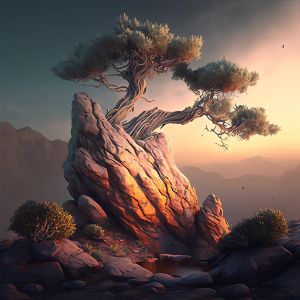This image, rendered in pixel art style, depicts a rugged landscape centered around a dominant, irregular-shaped boulder, which appears almost like a dog's howling mouth. Sprouting from the top of this craggy rock is a twisted, gnarled tree with two thick trunks, reminiscent of bonsai trees but considerably larger. The tree's branches are densely packed with leaves at the top. The foreground features stony ground interspersed with small bushes and a line of large rocks that seem to border a potential pool. In the distance, a dim mountain range runs along the horizon, under a moody sky. The sky itself transitions from dark blue on the left to a reddish-yellow glow on the right, suggesting a setting or rising sun.